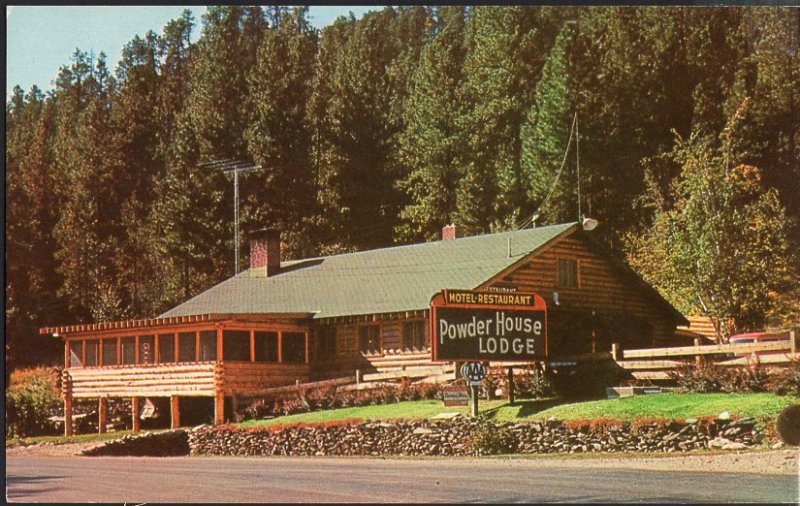In this vintage photograph, likely from the 1970s, we see the Powderhouse Lodge, an authentic wooden house that serves as a motel and restaurant. The lodge, which boasts a sturdy triangular roof equipped with a chimney and solar panel, is constructed entirely of timber, giving it a rustic charm. In front of the lodge, a well-maintained grassy area leads to a road. Prominently displayed near the road is a signboard with "Powderhouse Lodge" written in whitish-green text on a black background, while "Motel and Restaurant" is highlighted above it against a red backdrop. Additionally, an AAA sign is visible below. The picturesque setting features a mountain lush with trees in the background, enhancing the lodge's serene and inviting ambiance.